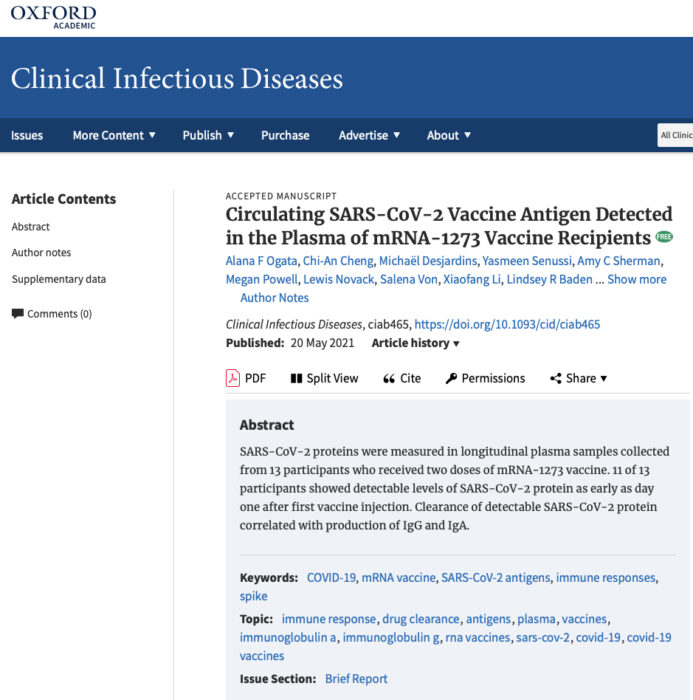This cropped screenshot depicts a webpage from Oxford Academic's website, specifically under the Clinical Infectious Diseases category. Dominating the top portion is a prominent blue header where "Clinical Infectious Diseases" is displayed in large white font. Directly below, a thick blue border contains navigation options labeled "Issues," "More Content," "Publish," "Purchase," "Advertise," and "About," with most featuring dropdown boxes to the right, though none are currently expanded.

The main body of the webpage, in stark white, begins with a sidebar labeled "Article Contents." Listed under this heading are categories such as Abstract, Author Notes, and Supplementary Data, with a "Comments (0)" section underneath. Adjacent to this sidebar is the abstract of a scientific paper, indicated as an "Accepted Manuscript" in small black letters at the top.

The title of the paper is "Circulating SARS-CoV-2 Vaccine Antigen Detected in the Plasma of mRNA-1273 Vaccine Recipients," followed by a list of authors. The name of the journal, "Clinical Infectious Diseases," along with a URL link, appears below the authors. Further down, the publication date is listed as "Published May 2021" and next to it is an "Article History" dropdown.

Options for interacting with the paper are provided, including "PDF," "Split View," "Cite," "Permissions," and "Share." The abstract of the paper is encapsulated within a blue box at the bottom. Finally, the page concludes with sections for Keywords, Topic, and Issues.